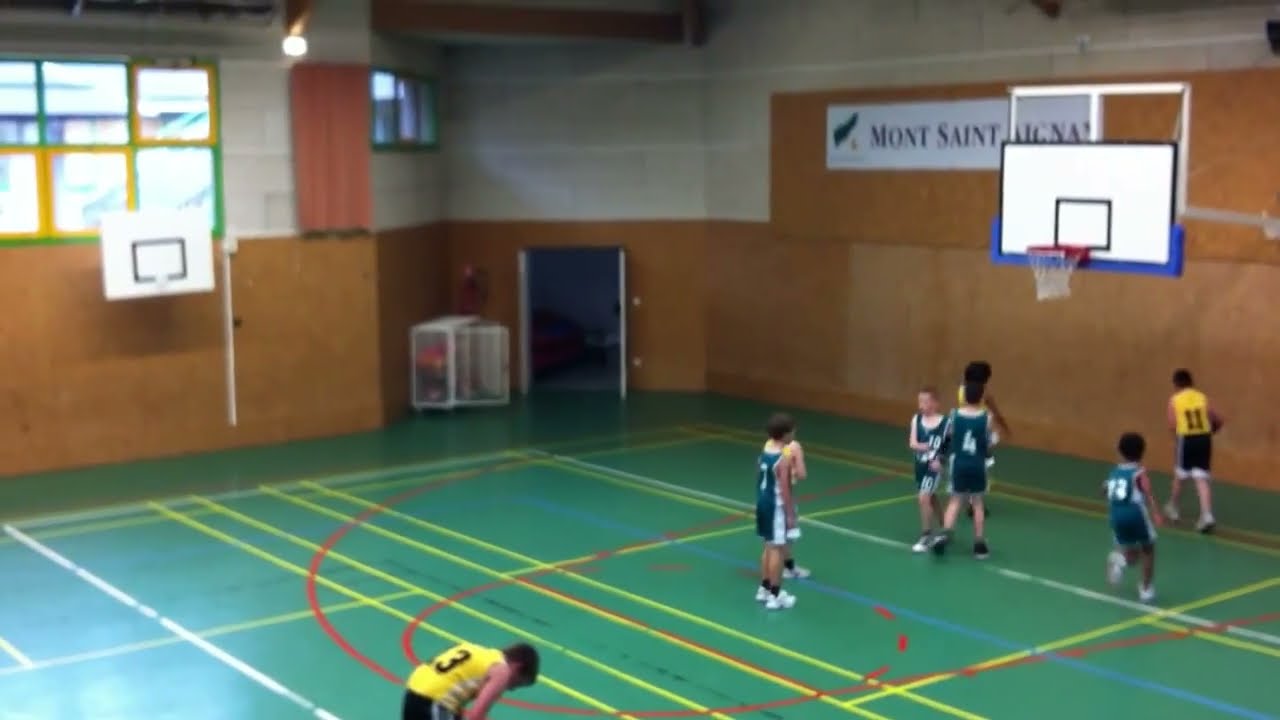This photograph captures a dynamic scene inside a basketball gymnasium where a game is underway between two teams of young boys, around 7 to 9 years old. The gym features a green floor accentuated with yellow and red stripes, and the walls are divided into a brown lower section and a white upper section. The basketball hoop, mounted on the wall, has a white backboard with blue trim. A banner above the hoop displays the school's name, "Mont Saint," though the rest of the text is obscured by the net.

The teams are distinguishable by their uniforms: one team is clad in green and white outfits with numbers 4, 7, 10, and 13, while the opposing team sports yellow tops, black shorts, and numbers 11 and 13. All the boys are wearing white or black sneakers. Details in the background include a blue door and a mesh wire cabinet, with windows visible on the left side. The image, while slightly out of focus, captures the energetic atmosphere of the game.